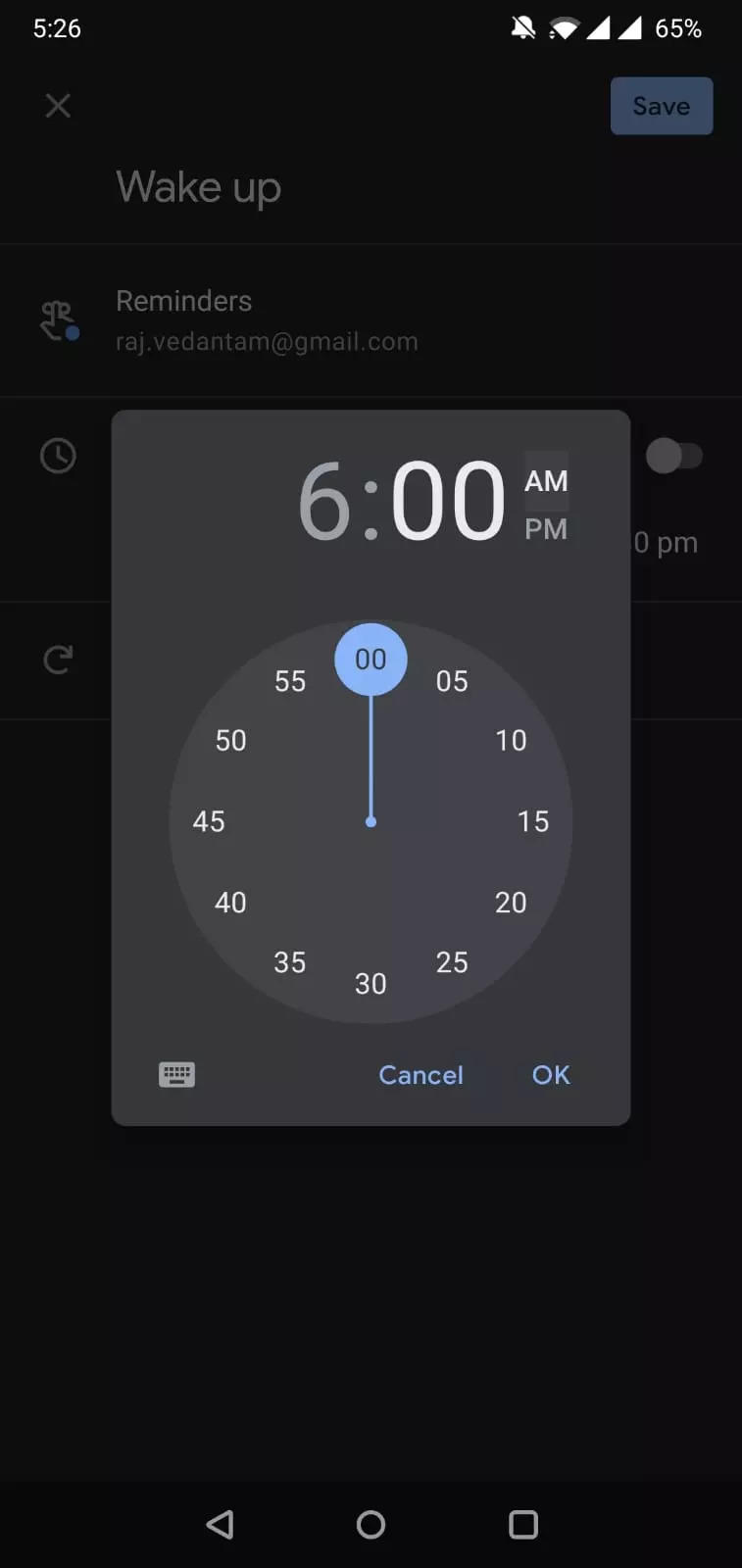This image depicts a smartphone screen showcasing an alarm clock app interface. At the top of the screen, the status bar displays the current time, battery percentage, and a notification bell icon. Dominating the screen is a pop-up for setting an alarm, showing "6:00 AM" with an option to switch to "PM." Surrounding the time are selectable circular increments in five-minute intervals, starting from "00" and going up to "55."

Below the circular clock interface, there are two prominent buttons: a blue "Cancel" button and a blue "OK" button. The main page of the app features the heading "Wake Up" above a reminder section. Within this section, an email address, "raj.ventum@gmail.com," is visible, presumably to send reminders to. The app appears to offer a variety of settings for creating alarms or timers, indicative of a standard clock app found on most smartphones.

At the bottom of the screen, three navigation icons are displayed against a black background: a white backward arrow, a white circle, and a white square, serving as the typical navigation controls. Despite the screen being predominantly black with white text, the interface includes several button colors, notably the blue "Save" button.